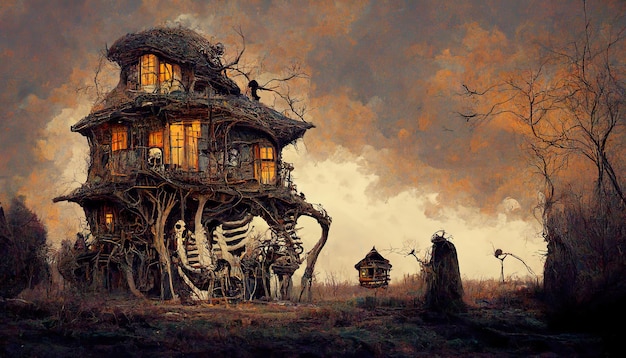The image depicts a haunting scene featuring a dilapidated three-story house, dark brown and seemingly constructed from a colossal tree intertwined with human skeletons. The house, bathed in an eerie orange glow from its large windows, appears to be suspended or supported by an enormous human skeletal structure, with a prominent skull and split ribcage facing forward. The roof is crafted from twisted branches, forming a domed, mushroom-like shape. Surrounding the house is a field of dead grass and wispy, leafless trees, contributing to the overall desolate atmosphere. The ground around the house is dark, while the ominous gray sky above has swirling streaks of orange, suggesting either nighttime or an impending storm. In the foreground, a small structure, possibly a doghouse or tombstone, adds to the creepy ambiance, and there is a figure approaching the house. Overall, the image exudes a profoundly haunted and eerie vibe, with every element enhancing its spooky nature.